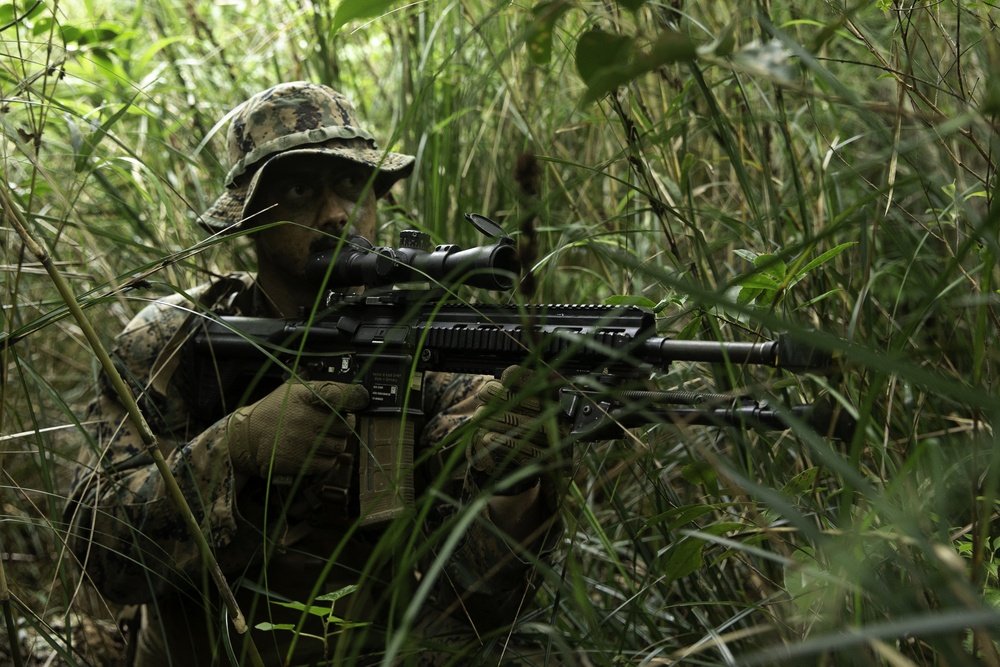In this striking, color photograph steeped in predominantly green tones, a soldier is captured amidst high vegetation, likely in a dense jungle or swamp area. The soldier is fully garbed in an olive green, camouflage-patterned uniform, complete with matching gloves and face paint designed to seamlessly blend into the lush surroundings. He stands surrounded by tall reeds that rise higher than his head, emphasizing the overgrown, wild nature of his environment. The soldier wears a brimmed hat, the brim slightly tilted up, giving a clear view of his intensely focused face as he looks to the right. 

He's holding an imposing assault rifle, equipped with a scope and featuring a large loading area, signifying heavy artillery. His finger is on the trigger and one hand steadies the barrel, suggesting a state of readiness and alertness. The photograph exudes a sense of tension and seriousness, underscored by the soldier's poised stance and unwavering gaze. There are no other figures or animals in sight, and no text distracts from the somber, solitary subject of the image.